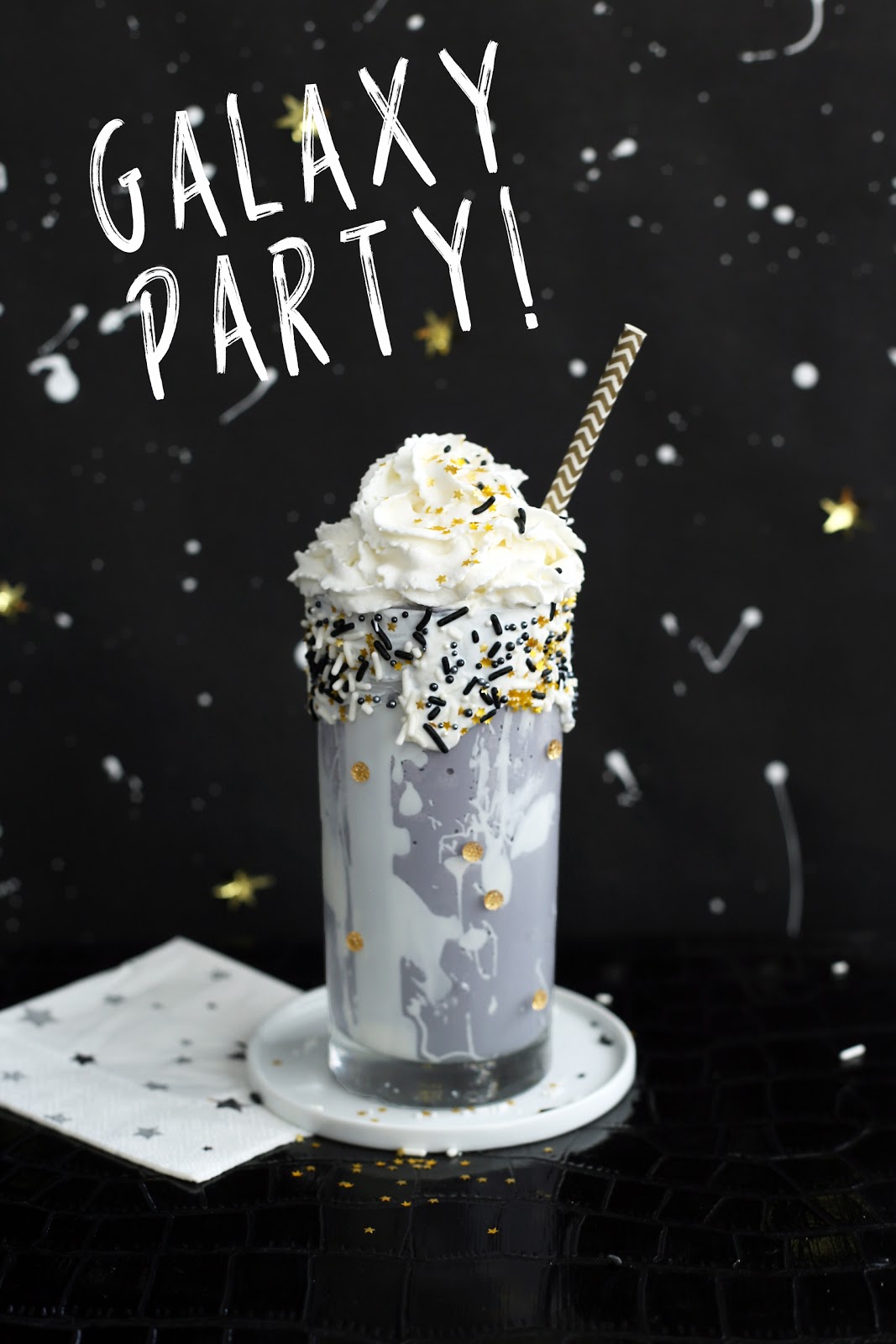This is a detailed photograph of a galaxy-themed milkshake, captured in a rectangular frame measuring approximately five by three inches. The focal point is a tall highball glass centrally placed on a white, thin saucer that rests on a black tabletop featuring an alligator-skin pattern. The milkshake itself is a purplish-gray color with white streaks, topped generously with white whipped cream. Scattered across the whipped cream are black, gold, and white star-shaped sprinkles, adding a celestial touch.

Emerging from the top right side of the glass is a gold-patterned straw with black and white stripes. Underneath the saucer lies a white napkin adorned with gray and black stars, enhancing the thematic decor.

The background is a dark gray or black wall embellished with white dots and yellow stars, some of which have streaks to appear like shooting stars. Two diagonal lines of text in uppercase white letters at the upper left corner declare "GALAXY PARTY!". The overall ambiance imparts an outer space atmosphere, perfectly marrying the whimsical and the elegant.